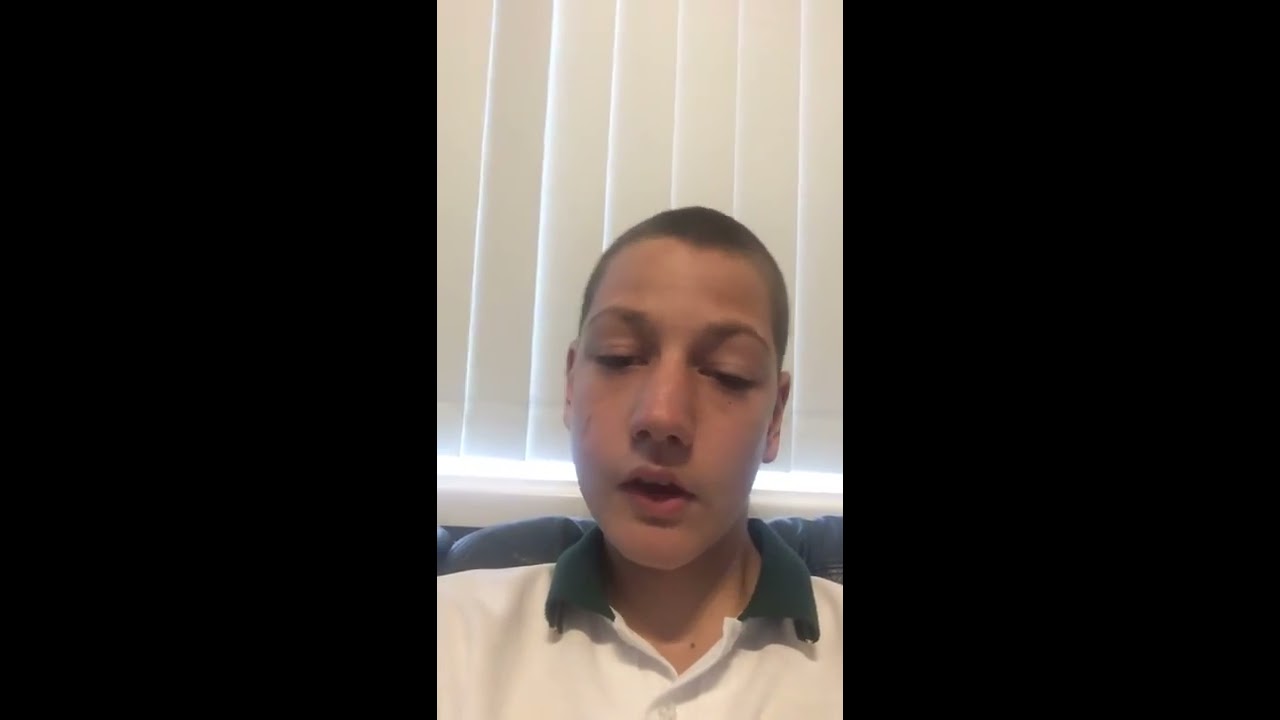The image captures a close-up of a young male, likely a teenager in his early teens, with a buzz cut or crew cut of dark brown to black hair. He is dressed in a white polo shirt with a green collar, with the top button unbuttoned and the second button fastened. His eyes are barely open, as if mid-blink, and his mouth slightly open with his head tilted slightly to the left. The background features a white windowsill with vertical white blinds and some light peeking through near the bottom. He appears to be seated on a couch, possibly leather, with black borders framing the left and right sides of the image. The photo is vertically oriented, suggesting it was taken on a cell phone. His expression and posture convey a sense of casualness.